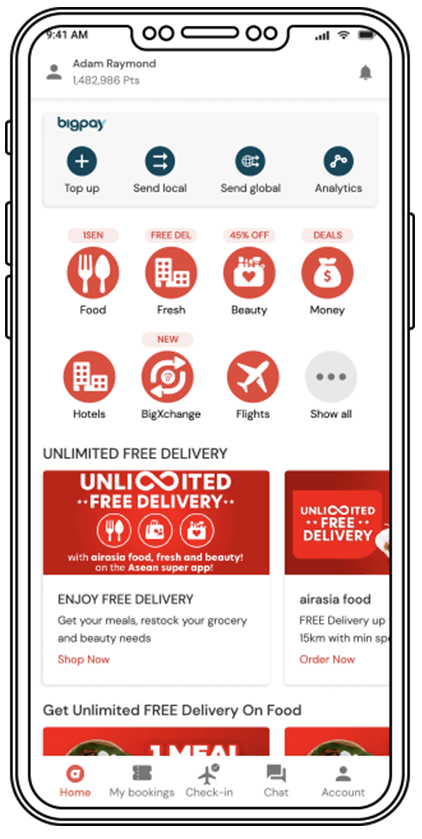Detailed Caption:

The image showcases a simulated cell phone with a white body outlined in black, giving it a digital, albeit somewhat amateur, aesthetic. The phone screen displays various elements against a white background. At the top, it shows the time "9:41 a.m." alongside typical smartphone icons like a battery icon, Wi-Fi symbol, and signal strength indicator.

Immediately below these icons, there is the name "Adam Raymond," accompanied by a small gray person icon representing a head and shoulders. Next to the name, the screen shows a score of "1,482,986 points" and a small bluish bell icon.

Further down, the phone screen transitions to a gray background with blue and black fonts. It features various options and actions:
- "Top Up" with a circular icon containing a plus sign.
- "Send Local" with a circle icon showing two white arrows.
- "Send Global" marked by a blue circle housing a small white globe.
- "Analytics" represented by three white circles.

Below these, there is a row of categories shown as red circles with white icons:
- "Food" featuring a fork and spoon icon.
- "iSend" without a specific icon detail.
- "Fresh," which has building icons and a label saying "Free DEL."
- "Beauty," represented by a little makeup bag with a heart icon and some brushes, along with "45% off" text.
- "Money," indicated by a bag of money icon and the word "Deals."
- "Hotels" with building icons, and "Big Exchange" featuring arrows in a circular pattern.
- "Flights" represented with an airplane icon, followed by a gray "Show All" option with dots.

At the bottom part of the phone screen, the text "Unlimited free delivery" appears in gray. The section highlights several red and white boxes proclaiming "Unlimited free delivery." This includes icons such as a fork and spoon, a small bag, and a makeup bag with a heart, with the text "AirAsia food fresh and beauty on the ASAN super app."

Further, it invites users to "Enjoy free delivery. Get your meals, restock your grocery and beauty needs," with a "Shop Now" button.

The footer of the screen includes various icons:
- "Home" with a red icon.
- "My Bookings" with a gray ticket icon.
- "Check-in" with a gray airplane icon.
- "Chat" featuring a gray text box.
- "Account" represented by a little person head icon.